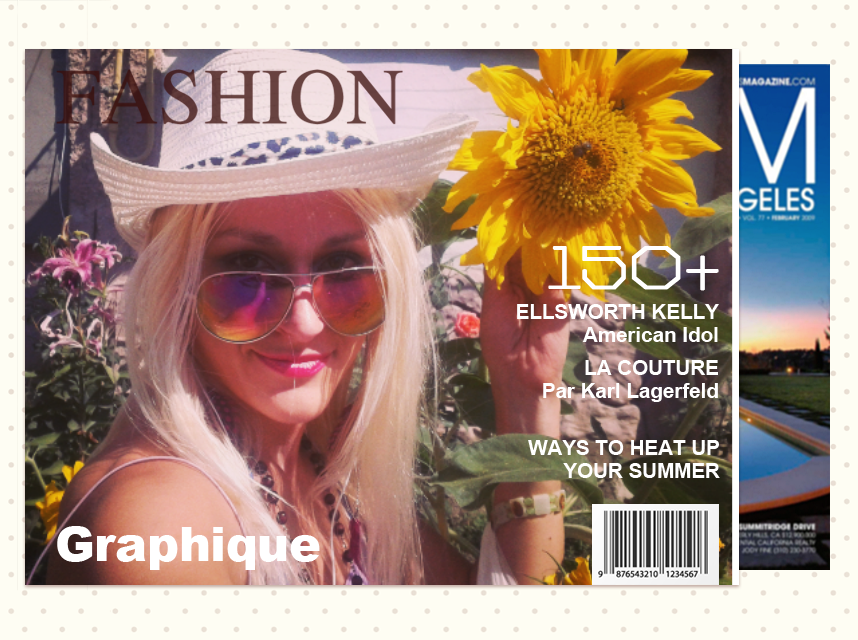This detailed image depicts a fashion magazine cover set against an off-white background with black polka dots. The focal point is a woman with long blonde hair, smiling, and wearing tinted sunglasses and a white hat. She is dressed in a sleeveless top and some jewelry, holding a large yellow sunflower in her left hand. The background includes green foliage. The title "FASHION" is displayed in brown uppercase letters at the top left, and "GRAPHIQUE" is written in white at the bottom left. On the right side of the cover, the text reads, "150+ ELLSWORTH KELLY, AMERICAN IDOL, LA COUTURE PAR KARL LAGERFELD, WAYS TO HEAT UP YOUR SUMMER," in white letters. A black and white barcode is situated at the bottom right. Partially visible is another magazine cover to the right, featuring a pool, a green field, and a blue sky, with the text "G-E-L-E-S," presumably for Los Angeles. This setup evokes a sense of summery, high-fashion elegance, with vibrant colors including tan, yellow, pink, purple, white, green, red, gray, and blue.